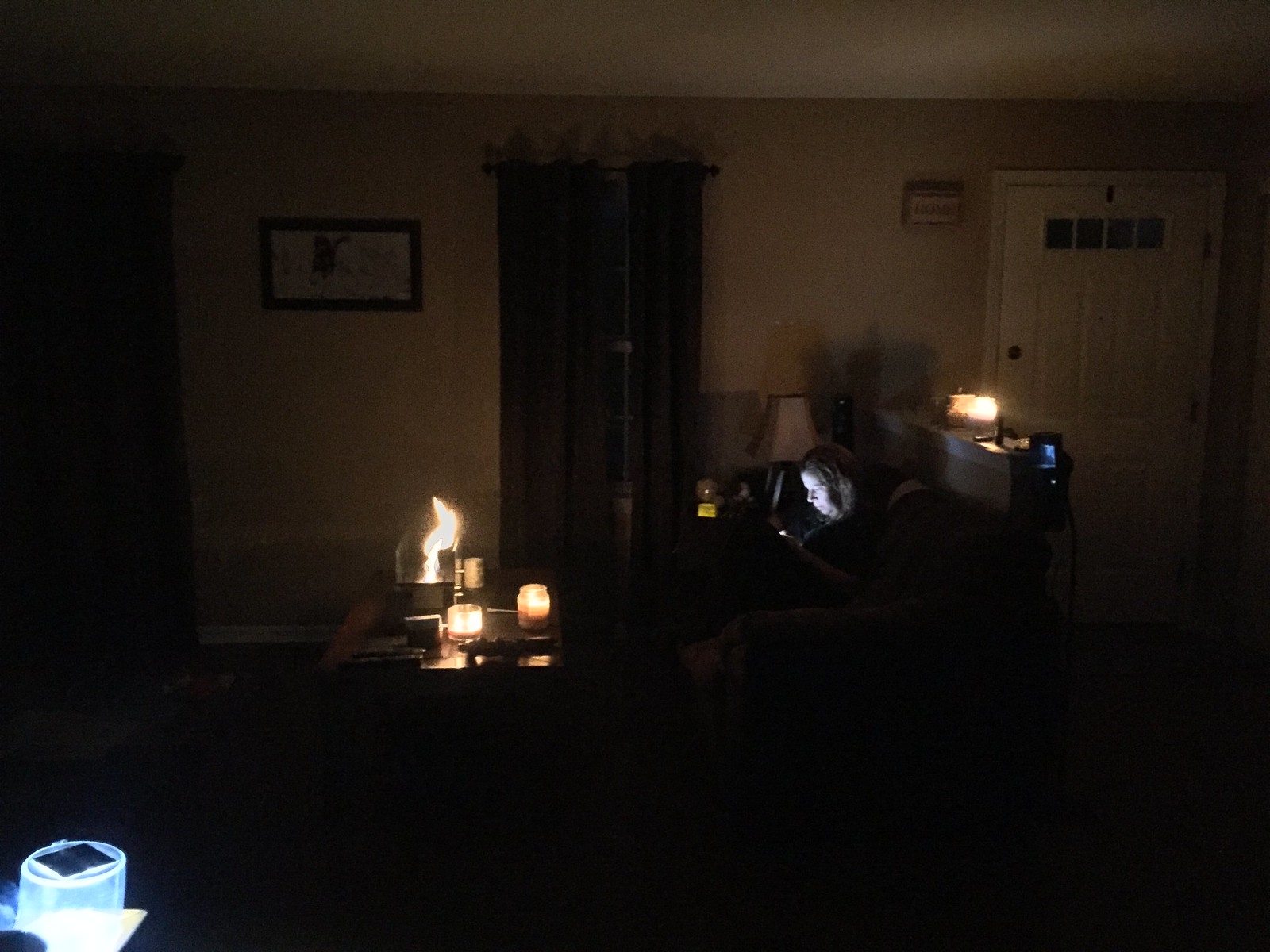In the dimly lit living room, the ambiance is set by the soft glow of multiple candles and salt lamps, casting a pinkish-red hue and a bluish-white light across the room. The lightly colored walls—potentially tan, white, or gray—are difficult to discern in the low lighting. A white door with four small windows occupies the far right, adjacent to a dividing wall that separates the living area. This wall also supports a candle or salt lamp, contributing to the warm glow. Centered in the room and framed by dark curtains covering a window behind her, a woman with long blonde hair sits on a couch or loveseat, her face illuminated by the light from her mobile device, which she is intently focused on. To her right stands an unlit lamp, while in front of her, a coffee table bears a collection of candles and salt lamps, further enhancing the cozy, intimate feel. A black-framed picture hangs on the far left of the wall, adding a touch of decor to the serene yet shadowy setting.